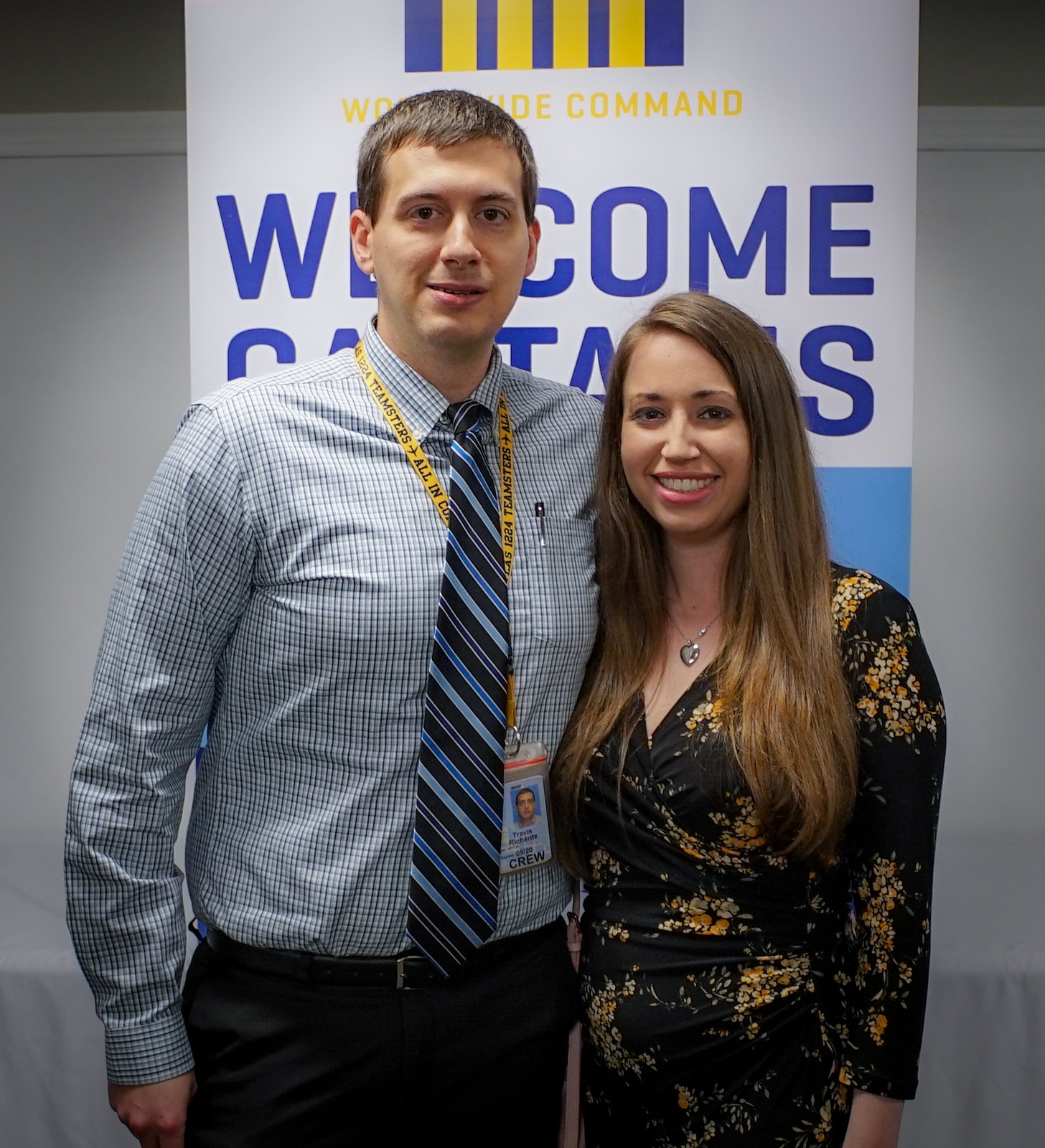In the color photograph, a man and a woman stand side by side in front of a sign with a white and blue background that appears to say "Worldwide Commander, Welcome Captains," though the text is not fully legible. The man, situated on the left, is dressed in a checkered shirt featuring shades of blue, white, and black, paired with dark pants. He accessorizes with a light blue and dark blue striped tie and a yellow lanyard carrying an ID badge that lists his name and crew. The woman to his right, with long brown hair, is attired in a black dress adorned with a floral pattern in various shades of yellow. She also wears a pendant necklace. The setting suggests a military-related event, and the background includes a gray wall.